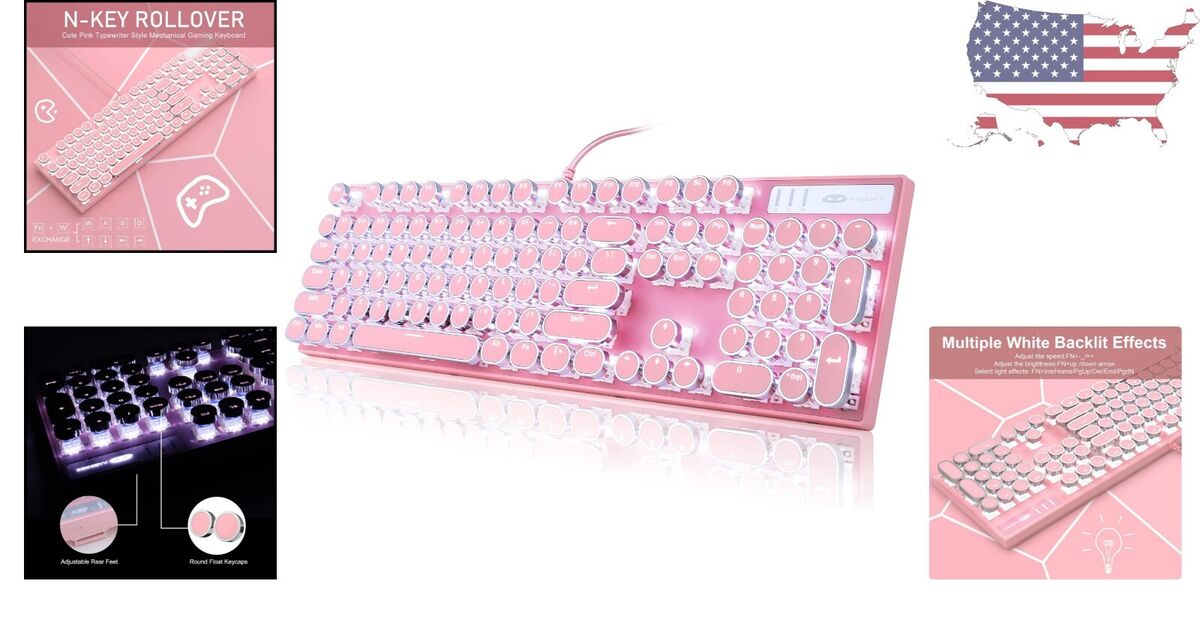This is a detailed advertisement image for a decorative pink keyboard with multiple white backlit effects. The central focus is a shiny pink keyboard, featuring a pink cord extending from the top and keys made from a shiny pink plastic with a clear or white edge around them, suggesting backlighting capabilities. To the left, there is a label reading "N-key rollover" accompanied by an image of the pink keyboard shown sideways. Below this, another image presents a black version of the keyboard illuminated against a dark background. To the right of the main keyboard, the text "multiple white backlit effects" is displayed. In the upper right-hand corner of the image, there is an outline of the United States filled with the American flag, indicating that the keyboard is made in the USA. The keyboard’s keys are notably round rather than the traditional square shape, adding to its unique, decorative appearance.